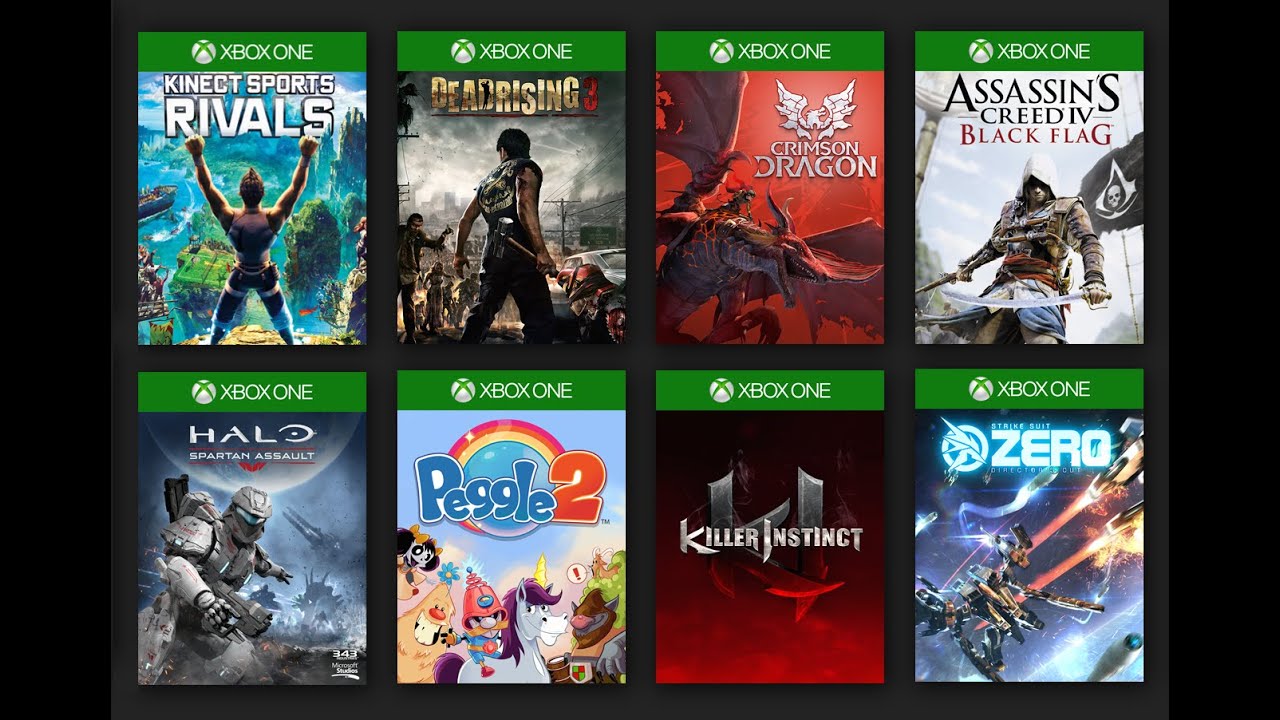The image features a black background showcasing the covers of eight Xbox One games, each cover marked with a green border and the Xbox One logo across the top. Starting from the top left, the first game is "Kinect Sports Rivals," displaying an athlete with arms raised in triumph. To its right is "Dead Rising 3," which depicts a character gripping a large metal hammer. 

Continuing right, the third game is "Crimson Dragon," spotlighting a bold red dragon against a matching red backdrop. The fourth game on the top row is "Assassin's Creed IV: Black Flag," featuring a rugged warrior brandishing swords in both hands, with a black flag adorned with a skull fluttering behind him.

Moving down to the second row, the first cover shows a composite of four game icons, with "Halo: Spartan Assault" in the lead, presenting a heavily armored soldier or robot. Next to it is "Peggle 2," a whimsical children's game featuring animated characters like a furry brown creature with big white teeth, a flower, a unicorn with a purple mane and golden horn, and another horned creature. 

Adjacent to it is "Killer Instinct," set against a predominantly red and gray background. The final game on the bottom right is "Strike Suit Zero: Director's Cut," which depicts what appears to be a robot or spaceship engaged in a fierce battle.